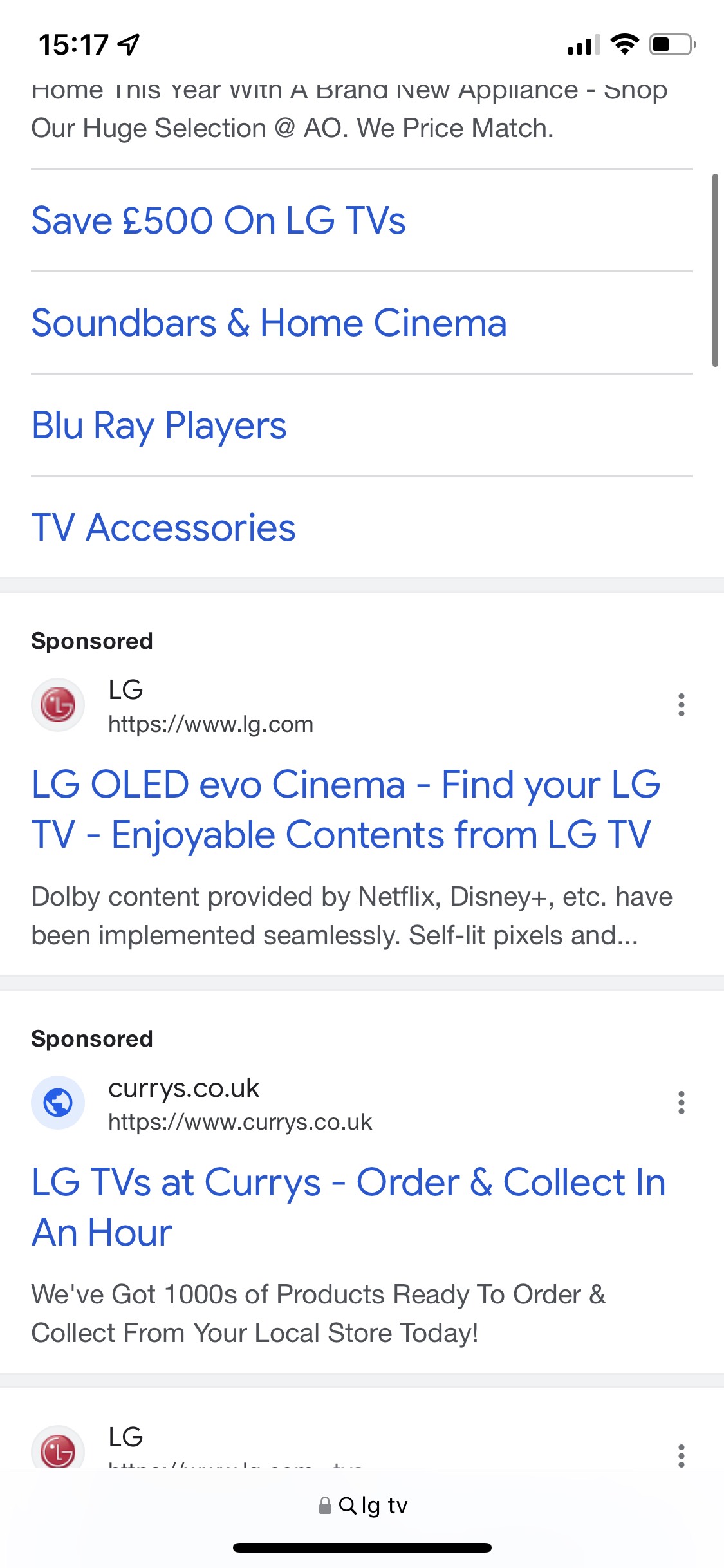**Detailed Caption:**

This image captures a mobile screenshot of a results page, predominantly showcasing promotional content related to LG products. At the very top, partially visible text reads "Save £500 on LGTVs, sound bars, home cinema Blu-ray players, and TV accessories," highlighted in blue text. Beneath this, the page specifies that the content is sponsored.

Just below, there is a recognizable red LG logo accompanied by the brand name "LG" and a URL link displayed as "https://www.lg.com". Following this, in blue text, the promotional tagline reads, "LG OLED Evo Cinema: Find your LG TV. Enjoyable contents from LG TV." Additionally, a functional feature is highlighted in black text, "Dolby content provided by Netflix, Disney Plus, etc., implemented seamlessly with self-lit pixels..."

Further down, the advertisement is noted to be sponsored by "Currys," and in blue text, it directs consumers to "LGTVs at Currys: Order and collect in an hour." Directly below, in black text, it reassures potential buyers with the message, "We've got thousands of products ready to order and collect from your local store today."

Another red LG logo appears towards the bottom of the screenshot, emphasizing the brand once more. Additional text indicating a time, "15:17," is visible in the top left-hand corner. Some more text is partially cut off but includes a promotional message about brand new appliances and price matching, with the identifiable symbol "@AO."

The entire image features a white background, common in mobile screenshots, emphasizing the clean and simple layout of the promotional content.